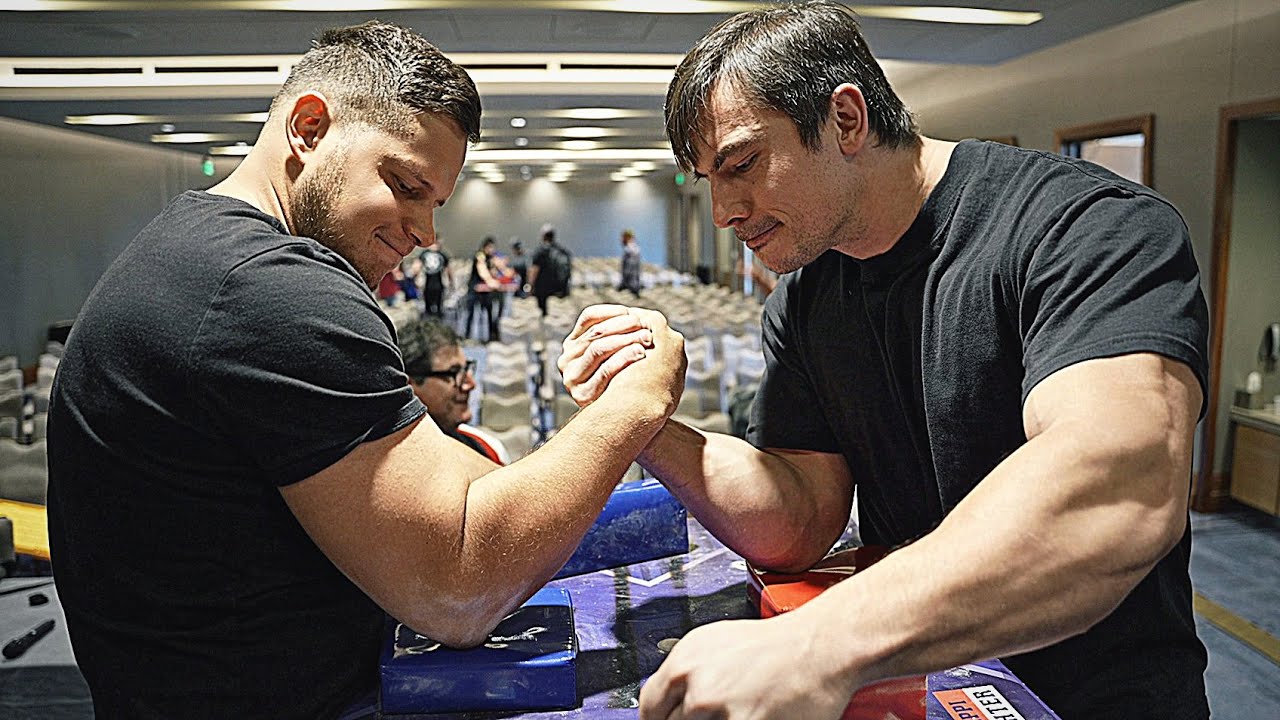The image captures an intense arm wrestling match between two muscular men, both dressed in black t-shirts. The man on the right sports black hair that is parted and hangs to the middle of his forehead, while his opponent on the left has a very short, brush-cut hairstyle and a beard but no mustache. Both men, who are white, have their right arms fiercely clasped together in the center of a table with a purple base, each gripping a peg with their left hands for support. The man on the right has a determined expression, emphasizing his bulging muscles, while the man on the left appears to be slightly leaning back with a grimace on his face. Behind the competitors is a seated man wearing black glasses, with short black hair, who seems to be disinterestedly looking off into the distance. The background is a blur of people, likely spectators, in what seems to be a convention room or stadium-type setting with fluorescent lights, adding to the bustling yet unfocused atmosphere.